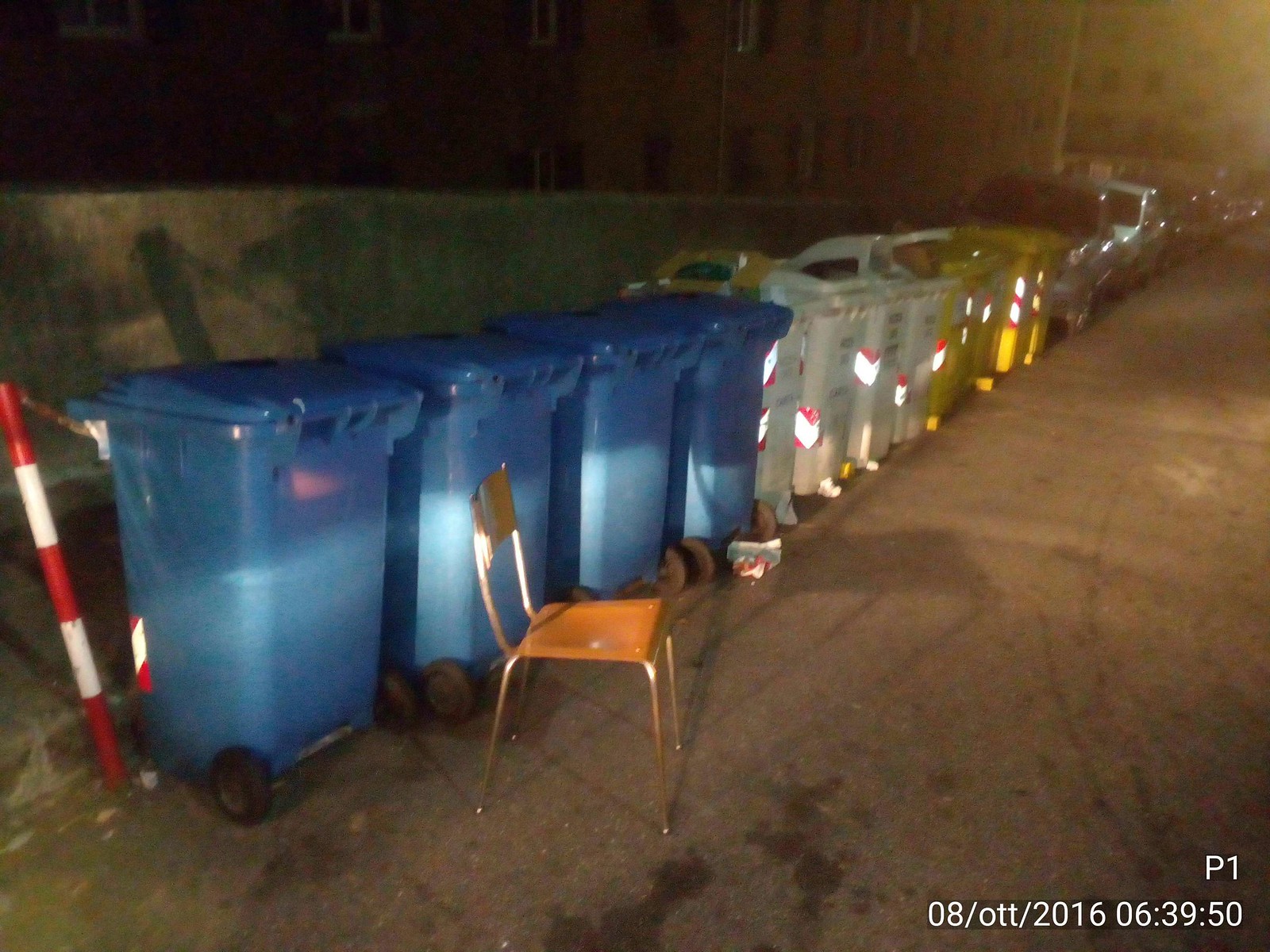The image depicts a shadowy and blurry night-time scene, reminiscent of security camera footage. It shows a row of large wheeled garbage bins—four blue, four white, and four yellow—lined up against a concrete wall. The bins are positioned on what appears to be a street or sidewalk, with parked cars including silver, white, and black vehicles seen in the background, along with apartment buildings with their darkened windows. To the left side of the bins stands a red and white striped pole, and near the blue bins is a wooden chair with metal legs. Notably, the bottom right-hand corner of the image bears text indicating it was taken on August 8, 2016, at 6:39:50, possibly PM. The overall scene has the eerie, low-quality atmosphere typical of surveillance footage.